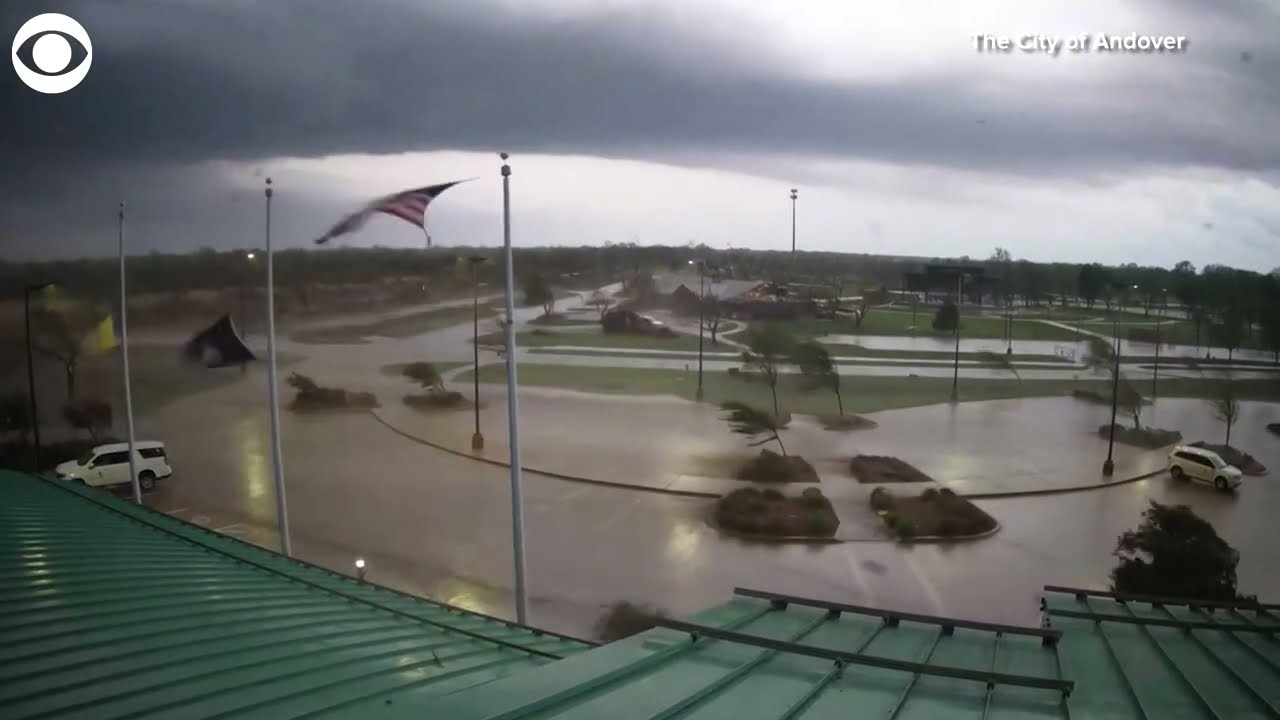The image depicts a stormy scene in the city of Andover, as indicated in white letters in the upper right corner. This photo, possibly taken with a wide-angle lens from the roof of a green metal building, captures an overcast sky filled with dark, gray clouds. The sun attempts to break through on the right side, but the overwhelmingly stormy weather dominates. Winds are strong, evidenced by trees bending and an American flag whipping violently on a flagpole. A white SUV is parked in a flooded parking lot below, surrounded by wet surfaces and reflecting the recent heavy rainfall. The view extends to distant main streets, houses, trees, and grassy fields, all appearing drenched and windblown, emphasizing the severity of the storm.